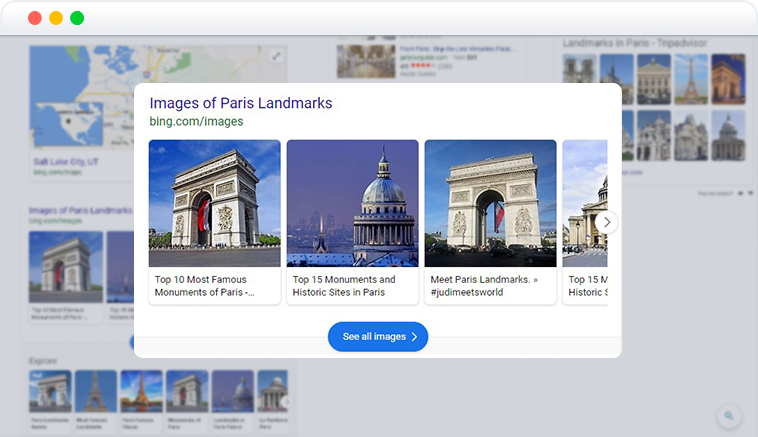This image depicts a horizontal rectangle frame. At the top, there are three dots in red, yellow, and green. The background appears blurred with indistinct images of various maps and travel locations, making it hard to discern specific details. Prominently in the center, there is a smaller horizontal white pop-up window. 

In the top left corner of the pop-up, written in a purplish hue, is the title "Images of Paris Landmarks." Directly below it, written in green lowercase letters, is "bing.com/images." 

The main content of the pop-up displays four partial vertical images arranged from left to right. The first image is labeled "The Top 10 Most Famous Monuments of Paris," the second says "The Top 15 Monuments and Historic Sites in Paris," and the third, labeled "Meet Paris Landmarks," additionally features the tag "#JudyMeetsWorld" below its description. The fourth image is partially cut off but includes a small arrow above it, indicating the possibility to scroll further to the right. 

Centered beneath these images, there is a turquoise horizontal oval button with the white text "See All Images."